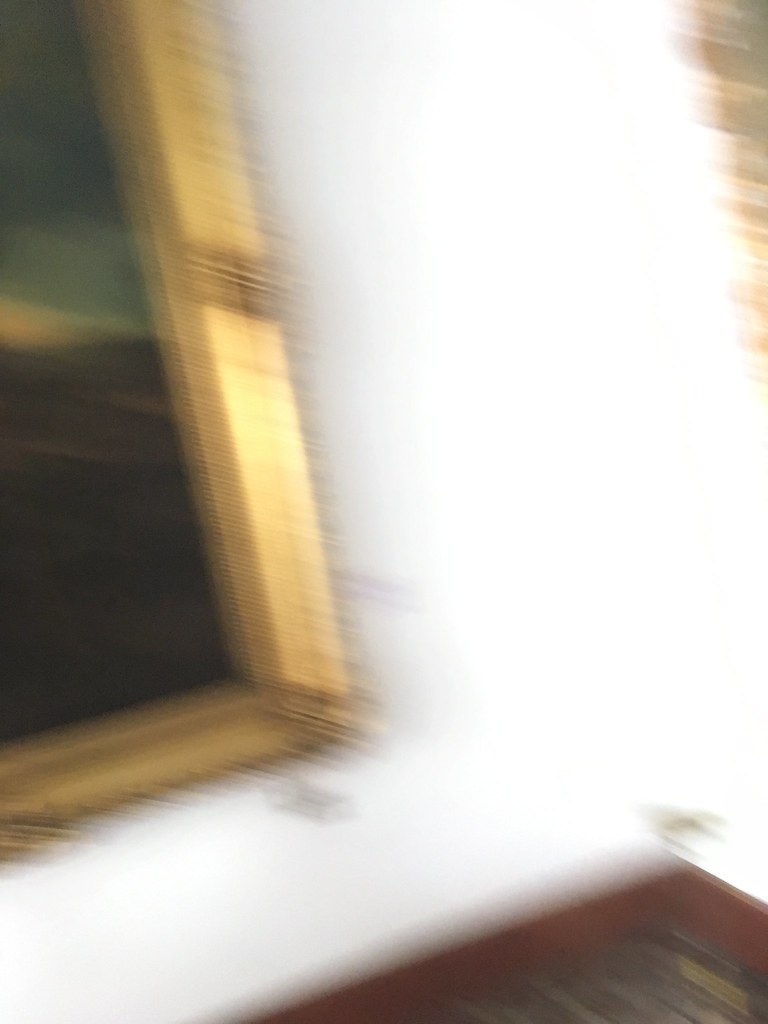The image depicts a well-lit, indoor setting, likely snapped inside a museum due to its noticeable details. The scene captures a blurred view of a white wall at the intersection of two corners. At the lower right, reddish-brown baseboards meet a floor characterized by greenish and silver tones with a shimmering effect, while elements of hardwood floor planks are evident. The left side of the image includes the edge of an elaborate gold-framed painting. Though heavily blurred, the painting seems to portray a scene with a darker upper section transitioning to lighter hues possibly depicting natural elements like a sky, ground, and perhaps mountains or clouds. The image is heavily blurred and overexposed, minimizing the clarity of finer details.